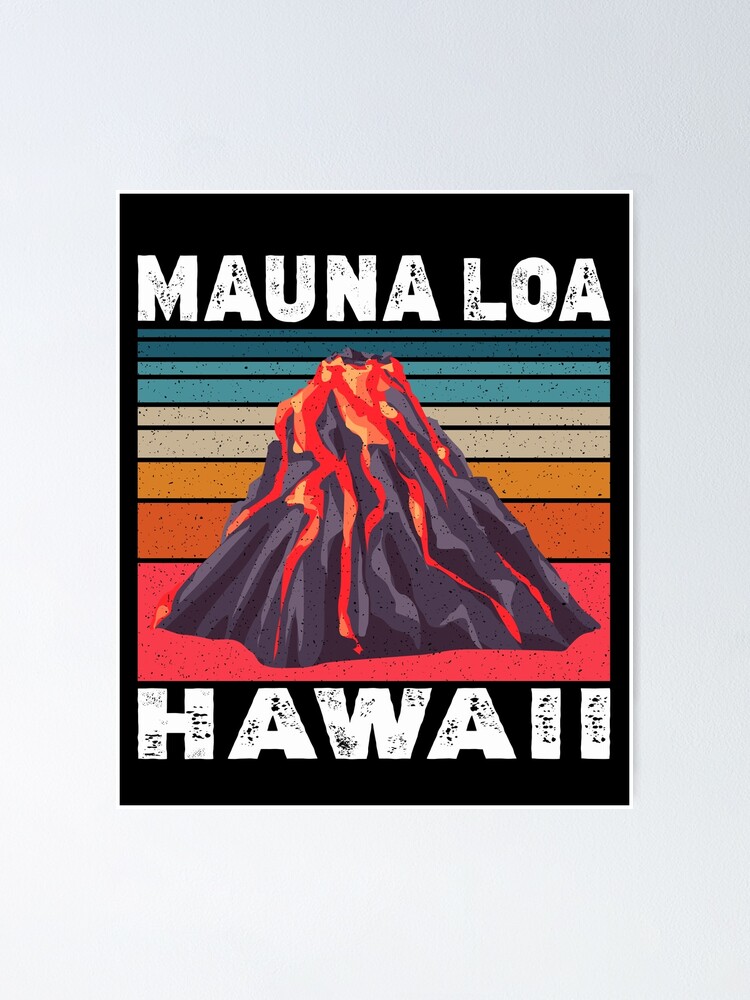On a minimalistic plain white background, the central poster artwork stands out with its deep black backdrop. Dominating the top of the poster, bold block letters spell out "MAUNA LOA" in all caps, rendered in bright white font speckled with black accents. Below this text, a vivid and somewhat playful drawing captures the essence of the Mauna Loa volcano. The volcanic rock is depicted in gray, with dynamic streams of orange-red lava flowing down its sides. Situated below the volcano graphic is another set of all-cap white letters, similarly speckled with black, proclaiming "HAWAII". The background behind the volcano is adorned with horizontal stripes that transition through a spectrum of colors: from shades of red and orange at the top, descending through tan, green, to a darker green as they reach the bottom. The overall image pulsates with energy and vibrancy, capturing the majestic and fiery essence of Mauna Loa, Hawaii.